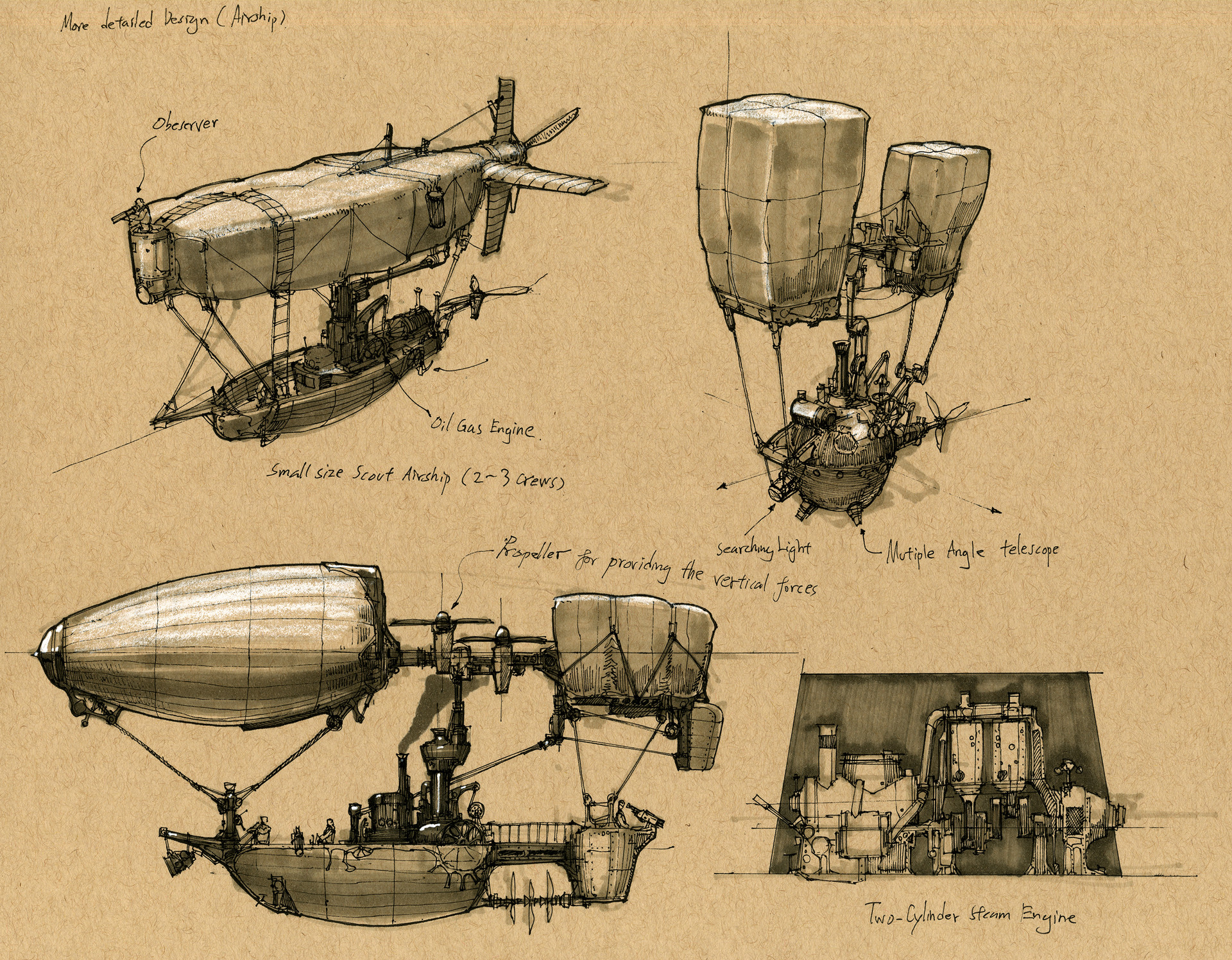This image is an intricate, old-fashioned mechanical illustration rendered on a dark beige, parchment-like background. The top left corner features a black script label that reads "More Detailed Design (Airship)." The image consists of four detailed sketches in black and brown ink.

1. The upper left drawing depicts a peculiar airship resembling a cross between a dirigible and a sailboat. This airship has a propeller at the back, rope ladders, and several components labeled: "observer," "oil gas engine," and "small size scout airship (two to three crews)."
2. To the right of the first sketch is another machine, marked with notations such as "searching light" and "multiple angle telescope," suggesting it might be another type of airship.
3. At the bottom left, a side view of a larger airship is shown. It includes a balloon-like structure on top and a boat at the bottom, with a label reading "propeller for providing the vertical forces." Several figures are visible onboard.
4. The lower right section features a drawing of a "two-cylinder steam engine."

The sketches are meticulously detailed and make extensive use of shading, all created in a black and ink style on the tan parchment, enhancing their vintage engineering aesthetic.